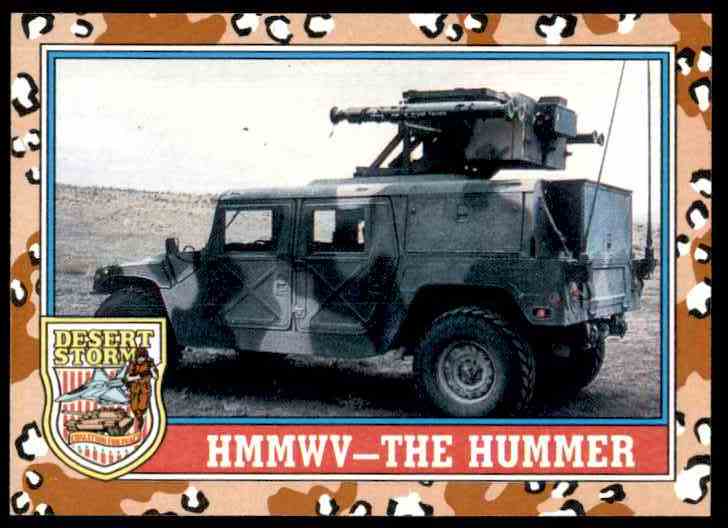This image captures a vivid, detailed portrayal of a military Hummer, specifically an HMMWV, prominently centered against a rugged terrain backdrop. The vehicle, painted in a desert camouflage palette encompassing shades of brown, green, gray, black, and white, is equipped with a weapon on top and features a rack that appears to hold luggage along with numerous bazooka-type rocket launchers. Two whip antennas extend upward from its rear, emphasizing its battle-ready state. The setting includes a stark white sky, enhancing the vividness of the Hummer's outline and its environment, which is clearly a desert landscape. The photograph is bordered by a distinctive brown desert camouflage frame with a black outline, adding a sense of depth and military aesthetic. At the bottom left of the frame, the emblem logo marked "Desert Storm" underlies the historical reference of the vehicle. The bottom center of the image includes the text "HMMWV - The Hummer." This setting suggests the image is an evocative piece, possibly displayed in a military museum to commemorate past military exploits and machinery.